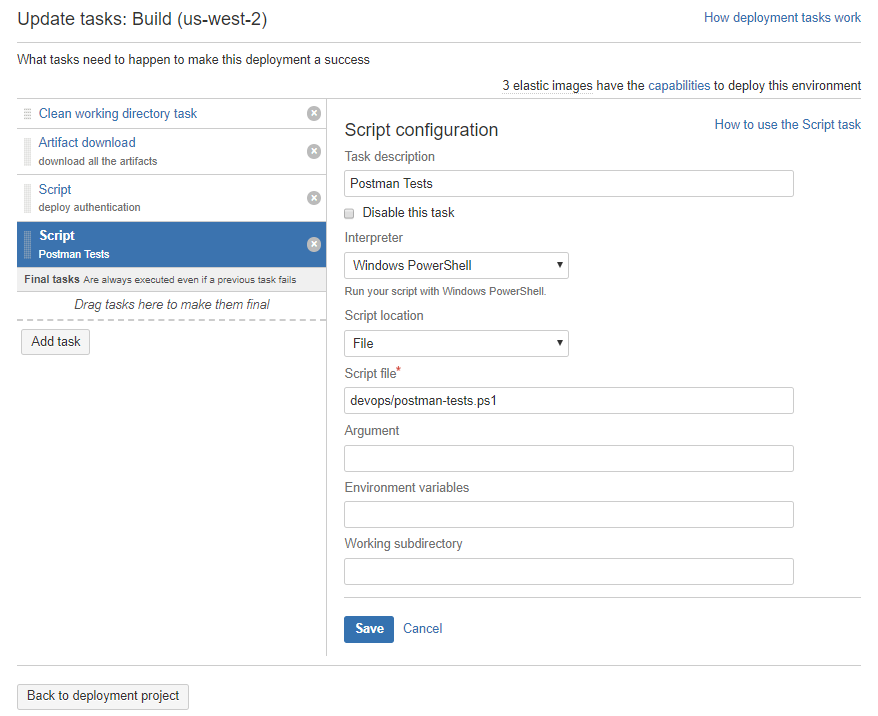The image depicts a detailed interface of a website dedicated to script deployment. 

At the top-left corner, a prominent heading reads "Update Tasks (build, US-West-2)" while the top-right features a smaller, blue-font hyperlink labeled "How deployment tasks work." This clickable link provides users with additional information on deployment procedures.

Below the heading, a section outlines the tasks required for a successful deployment. On the left-hand side, a list of items, each marked with an 'X', includes:
1. Clean Working Directory Task
2. Artifact Download
3. Script
4. Script (a different type of script)

This sequence is categorized under "Final Tasks." An 'Add' button is prominently displayed, allowing users to incorporate additional tasks into this section as necessary.

On the right-hand side, the interface dynamically displays detailed information pertaining to the selected task from the left-hand list. For instance, among the two scripts mentioned, the second one titled "Postman Tests" is highlighted in blue. Consequently, the right-hand pane provides comprehensive configuration details for this script, such as the task description, interpreter, script location, and the actual script file.

The organized layout and intuitive design effectively guide users through the deployment process, ensuring all functional aspects are clearly outlined and accessible.